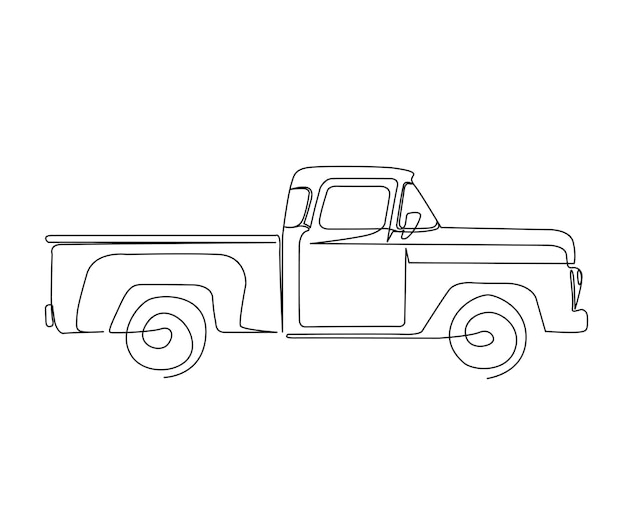This image showcases a simplistic, digitally-created line drawing of an old-style box truck with a flatbed. The black line, rendered on a white background, forms a continuous and rounded outline of the truck, giving it a soft and approachable appearance. The truck design includes several identifiable features: a single cabin likely designed to seat two to three people, circles for the tires, and connected squiggly lines. Notable details such as front and back lights protrude from the truck, and windows are present on the front windshield, back of the cabin, and door. Additionally, a side mirror is visible near the front door, which intriguingly lacks a handle. The overall simplicity and cohesive line work suggest that this image might serve as an icon or a digital representation found online.